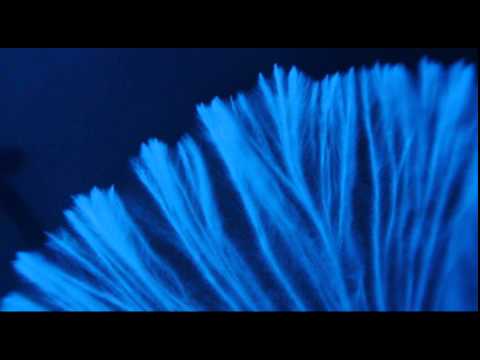The image features a striking, organic-looking structure resembling a fan of white, stringy threads or a feather-like, fractal pattern. This pattern is illuminated in light blue, creating a soft glow that contrasts with the very dark blue to navy blue background, which becomes slightly lighter towards the left edge. The threads extend unevenly and form a semi-circular archway, giving the impression of a delicate sea creature, possibly a coral or sea plant. The background includes subtle elements that might resemble rocks, adding to the underwater atmosphere. Encapsulated by black bars at the top and bottom, the widescreen format enhances the immersive depth of this ethereal scene.